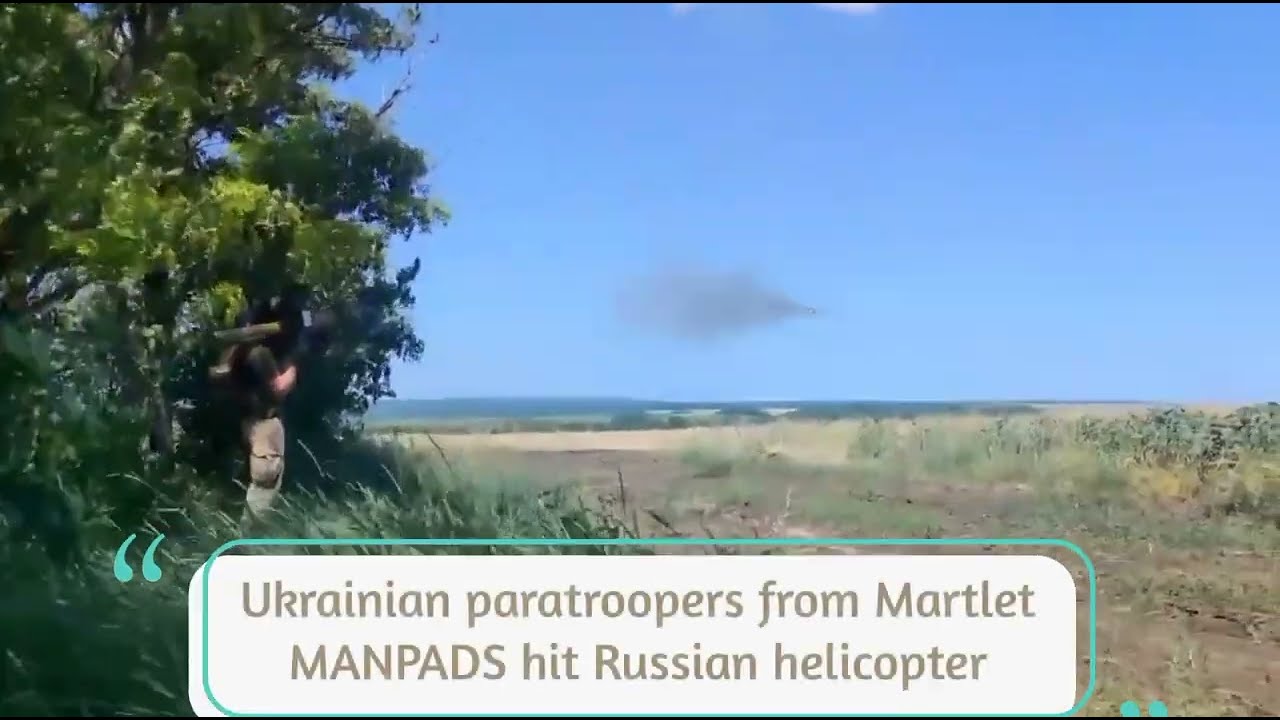A photograph captures an expansive field under a blue sky with distant green hills or mountains. The field is characterized by tall green grass and patches of brown grass interspersed with a dirt road running through it. On the left side of the image, a man stands partially obscured by foliage, holding a camouflaged rocket launcher on his right shoulder. He wears a green fatigued shirt and tan pants. His stance is strategic among the thick grasses, with a prominent tree to his left. Dominating the sky, a gray cloud of smoke trails from a rocket he appears to have just launched, suggesting a recent explosion. An overlaid caption at the bottom center of the photograph reads, "Ukrainian paratroopers from Martlet ManPADS hit Russian helicopter." The image is bordered by a thin black pinstripe at the top and bottom, and a blue-outlined rectangle with blue quotations is positioned just above and to the right of the caption.